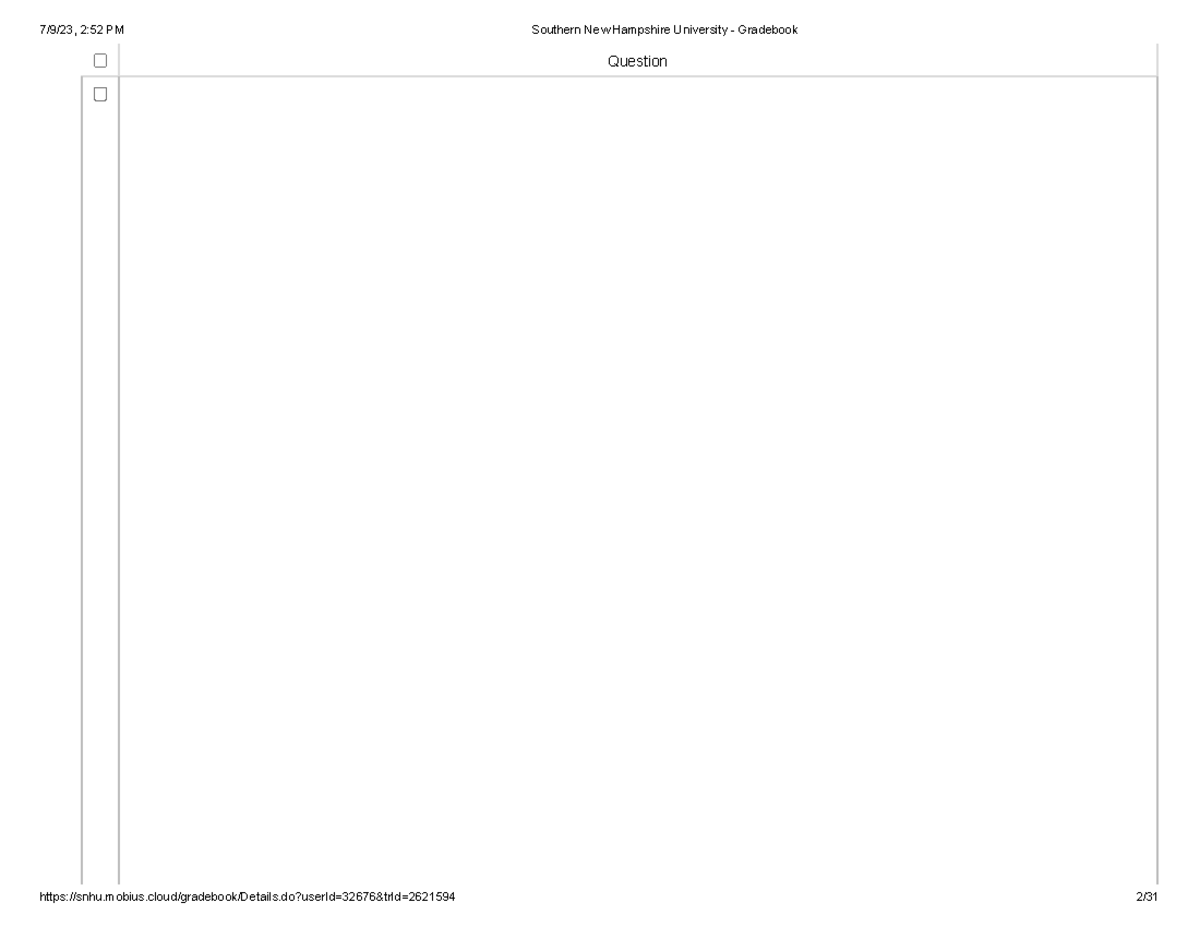The image displays a digital gradebook from Sullivan New Hampshire University. At the top of the image, the text "Sullivan New Hampshire University, Grade Book" is prominently displayed. In the top left corner, the timestamp "7/9/23, 2:52 PM" is visible. Below the timestamp, there are two rectangular boxes stacked vertically, and there is a horizontal line extending to the right and below these boxes.

On the left side of the image, a larger vertical rectangle is outlined, dividing two unchecked boxes positioned on the left and right sides. The bottom box aligns with the top of this vertical rectangle. Towards the right side of the image, the rectangular outline stops partway, replaced by a horizontal border that extends upwards past a central question area, protruding slightly above the horizontal line.

At the very bottom left of the image, there's a URL in black text. To the right of the URL, it reads "2/31." The full URL displayed is: "https://snhu.mobius.clouds/gradebook/details.do?userID=32676&TRLD=2621594".